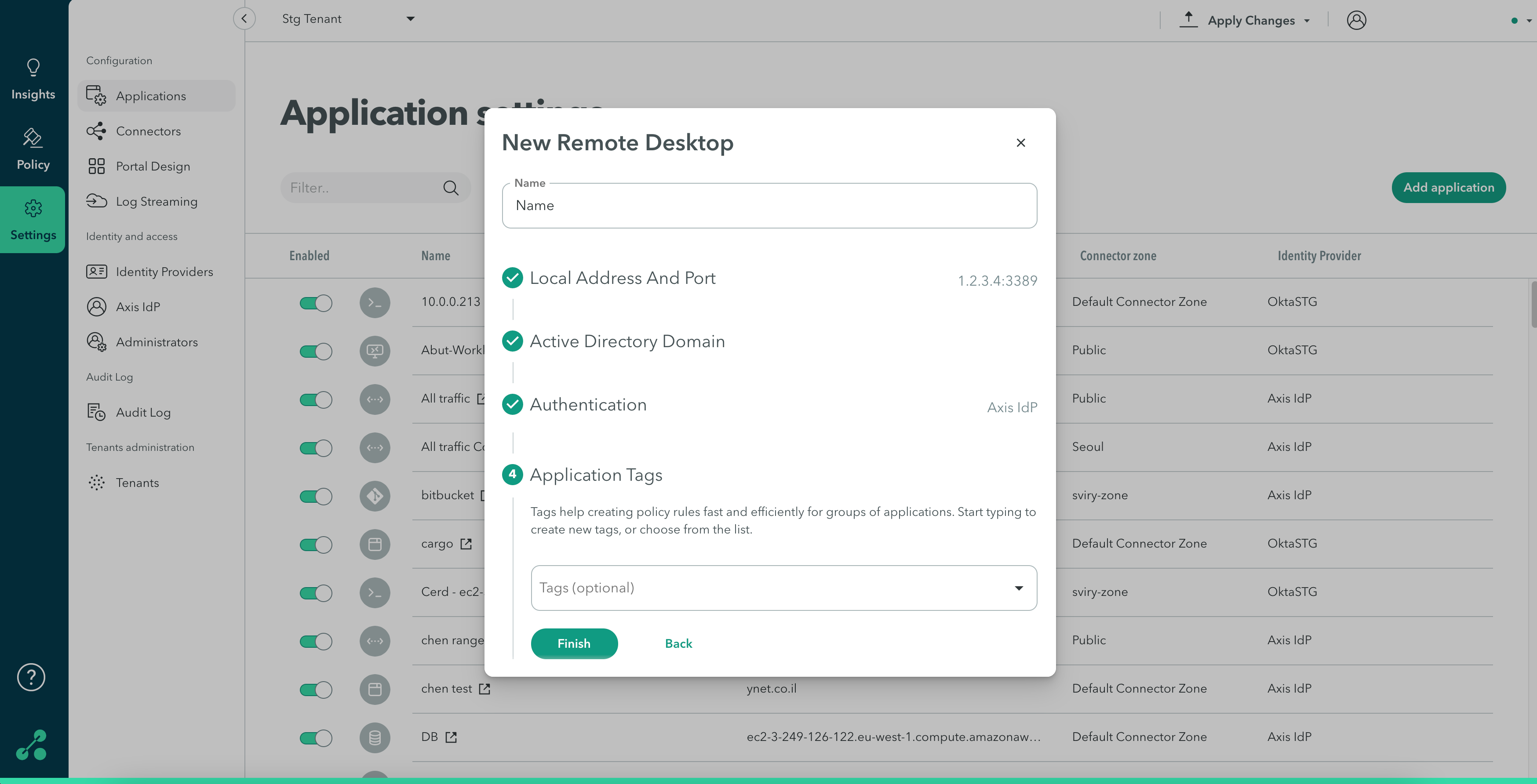The image depicts an interface layout of a software application. On the left side, there's a vertical menu displaying various options in sequence: "Insight," "Policy," and "Settings" highlighted in green. Adjacent to this menu, horizontally listed are options such as "Applications," "Connection," "Portal Design," "Log," and "Streaming." Below these options, the terms "Identity," "Providers," "Administrators," and "Audit Log" are visible, followed by the label "Tenants" at the bottom of the section.

In the center of the screen is a white panel titled "New Remote Desktop." This panel includes fields and options for setting up a remote desktop connection. The user is prompted to enter a name, a local address, and a port, with the sample entry for the latter displayed as "1.2.3.4:3389." Additional fields include "Active Directory Domain" and "Authentication," followed by a section labeled "Application Tags." There is guidance text explaining that tags help with creating policy rules and efficiently grouping applications, alongside a search bar to find or select tags from a drop-down list.

At the bottom of this panel, two buttons are highlighted: "Finish" in green, indicating it is the next step, and "Back" to navigate to the previous screen. Above this central panel, the interface also displays the heading "Application Settings" with an option to "Add SPCI Specification."